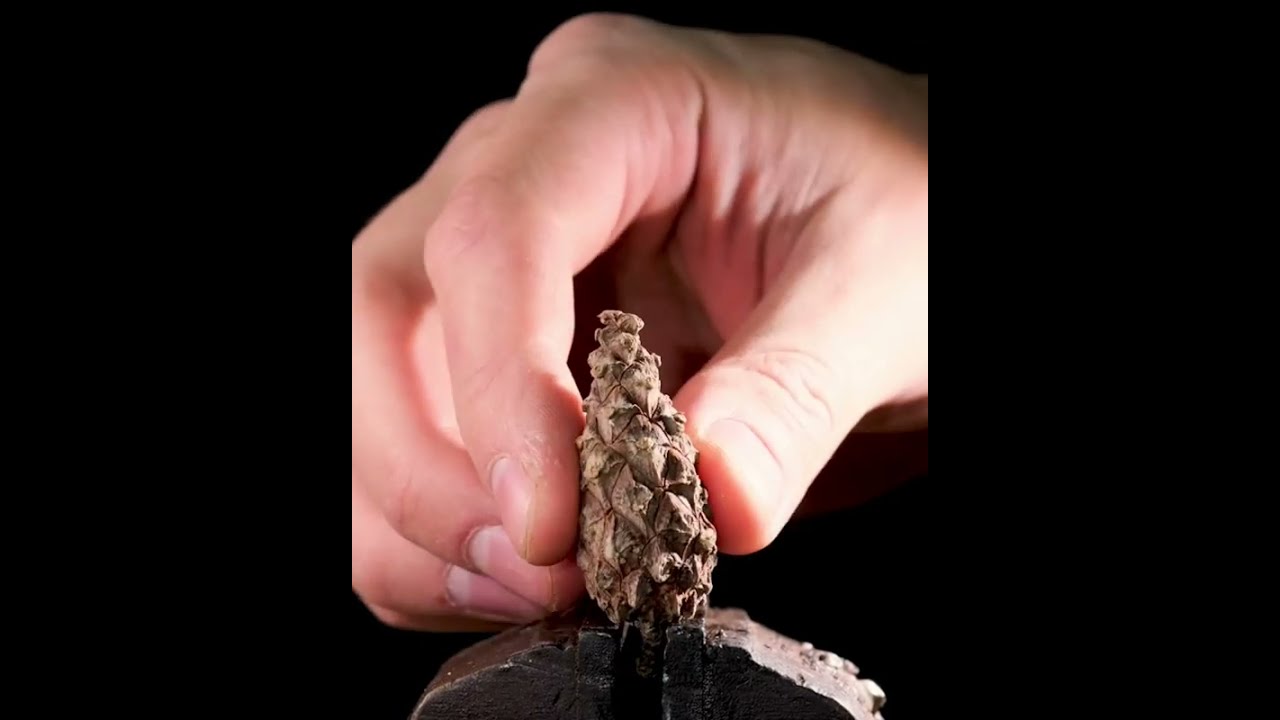Against a stark black background, the image features a close-up of a Caucasian person's right hand, with the thumb on the right and the index finger on the left, delicately pinching a small, bumpy object that resembles an acorn but is notably smaller. The object's surface is textured with sharp, ridge-like protrusions, akin to tiny shark teeth. It narrows towards the top and is held steady in a vintage, rust-colored vice clamp, barely visible in the lower part of the image. Flanking the hand and object on either side are two solid, black vertical bars, adding a geometric contrast to the organic forms. The lighting in the image highlights the thumb area, casting the left fingers and part of the object into shadow. The object also features what appears to be brown, leaf-like extensions at its base, spreading outward to the left and right.